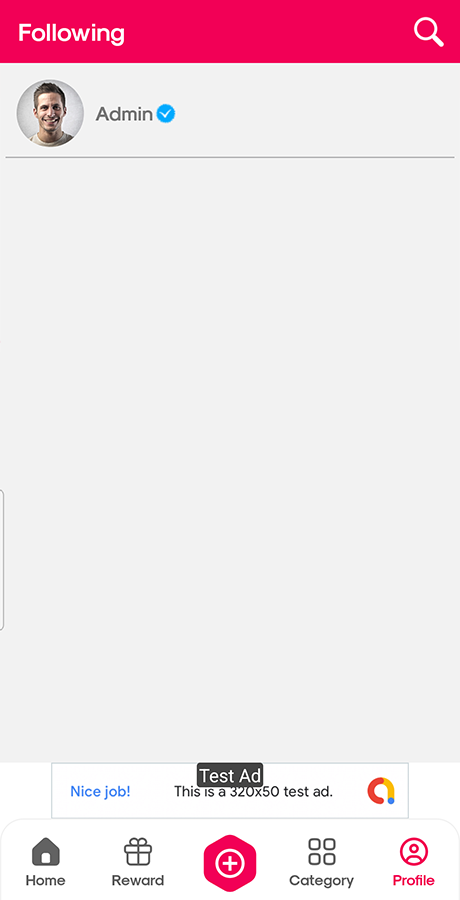The image features a test advertisement displayed on a mobile application interface. The top section of the screen includes a "Following" label and a search bar. Below that, there is an image of a male, likely in his 30s, with brown hair and a blue verification checkmark. He appears to be Caucasian. 

To the right of the man's image, there is an incomplete circular icon with segments in red, yellow, and blue, suggesting a logo without any identifying text. Beneath these elements, ample blank space is noticeable, likely intended for ad placement, accompanied by the text "Nice job."

The screen dimensions mentioned are 320 by 50 pixels, indicating the ad's size. At the bottom of the interface, there are navigation icons for Home, Reward, Category, and Profile. The Home icon is the traditional house symbol; the Reward icon resembles a gift box, and the Category icon consists of four small squares. The Profile icon, highlighted in magenta, suggests the current section in view.

Overall, this test ad appears to evaluate ad placement and formatting on a social media-like platform, with design elements akin to those seen on Facebook or Instagram.